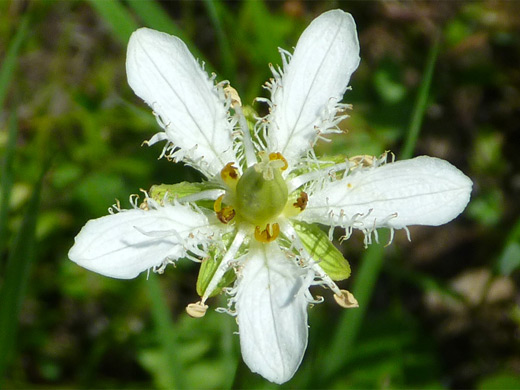This outdoor image captures a high-definition, top-down view of a delicate white flower, prominently featuring five petals adorned with wispy, feather-like hairs. The petals exhibit subtle green streaks, leading to a central core that is predominantly green with hints of yellow. The background, filled with blurred greenery, sharply contrasts the flower, making its fine details stand out. The photograph is horizontal and rectangular, emphasizing the intricate textures and colors of the flower itself.